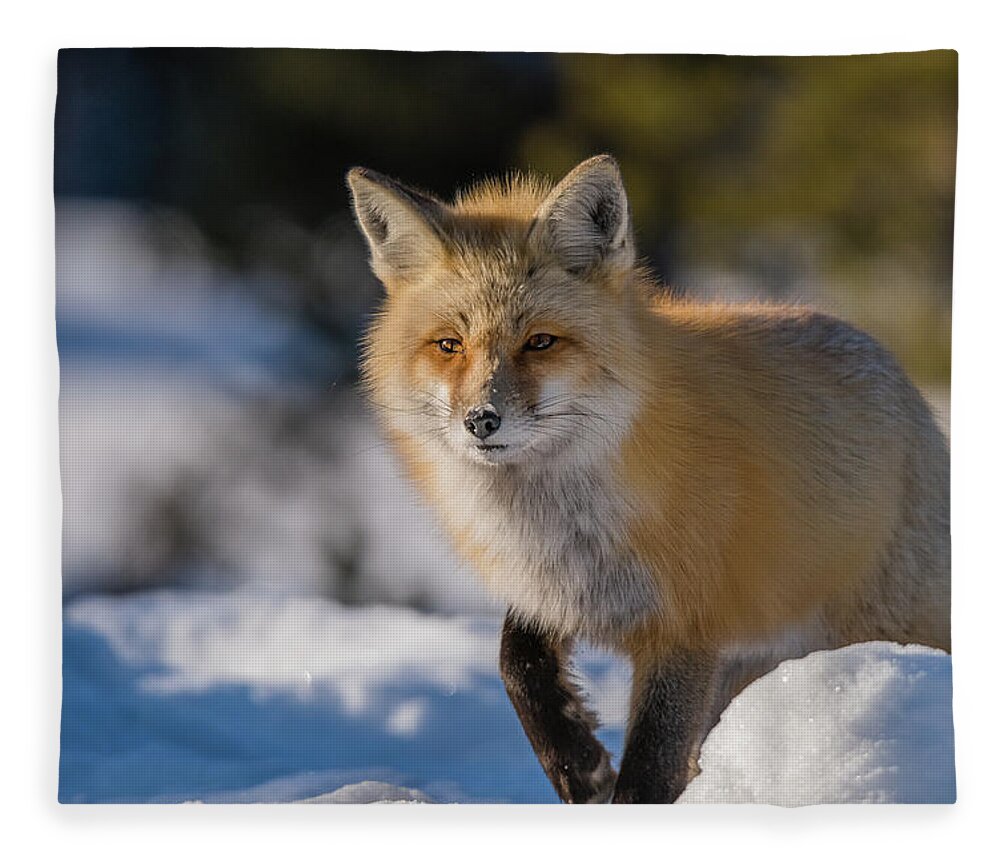In this outdoor image set in a snowy landscape, we observe a small fox, likely a baby red fox, traversing the snow-covered ground. The fox's coat is a mix of light reddish-brown and white hues, with darker fur accentuating its legs and various spots across its body. Its fur appears fluffy and stands up, giving a textured, natural look. The fox's eyes are brown, accompanied by a black nose and mouth. Sunlight illuminates the scene, causing the snow to glisten and highlighting the lighter shades of the fox's fur. In the blurred background, green trees and possibly distant mountain tops can be discerned. The fox, appearing somewhat curious or in search of something, gazes slightly off to the side of the camera, adding a sense of inquisitiveness to its demeanor.